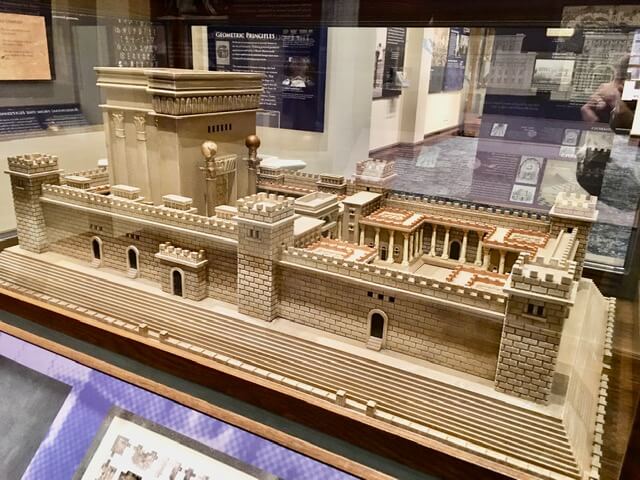The photograph captures a detailed, three-dimensional model, likely of an ancient, significant building, possibly resembling a temple in Jerusalem, enclosed within a plexiglass case set in a museum. The model represents an elaborate, large structure surrounded by fortified walls with six lookout towers adorned with trim. Its architecture includes arched openings that serve as entrances, leading inside to columned and sheltered areas, as well as open courtyards. The focal point of the model is a substantial rectangular building with two prominent gold columns, suggesting it could be a tomb, a church, or a special ceremonial site. The structure is rendered in a bleached clay color with intricate ramparts and access points like doorways and fortifications on the corners and middle of the walls. The model is meticulously detailed, with a green felt base and wooden lining, angled for optimal viewing. Surrounding exhibits and descriptions are visible in the museum's well-lit setting, with additional texts and images, although unreadable, providing further context. Reflections in the glass, including a hand, indicate someone examining the exhibit. The clarity of the image highlights the brightness and cleanliness of the museum environment.